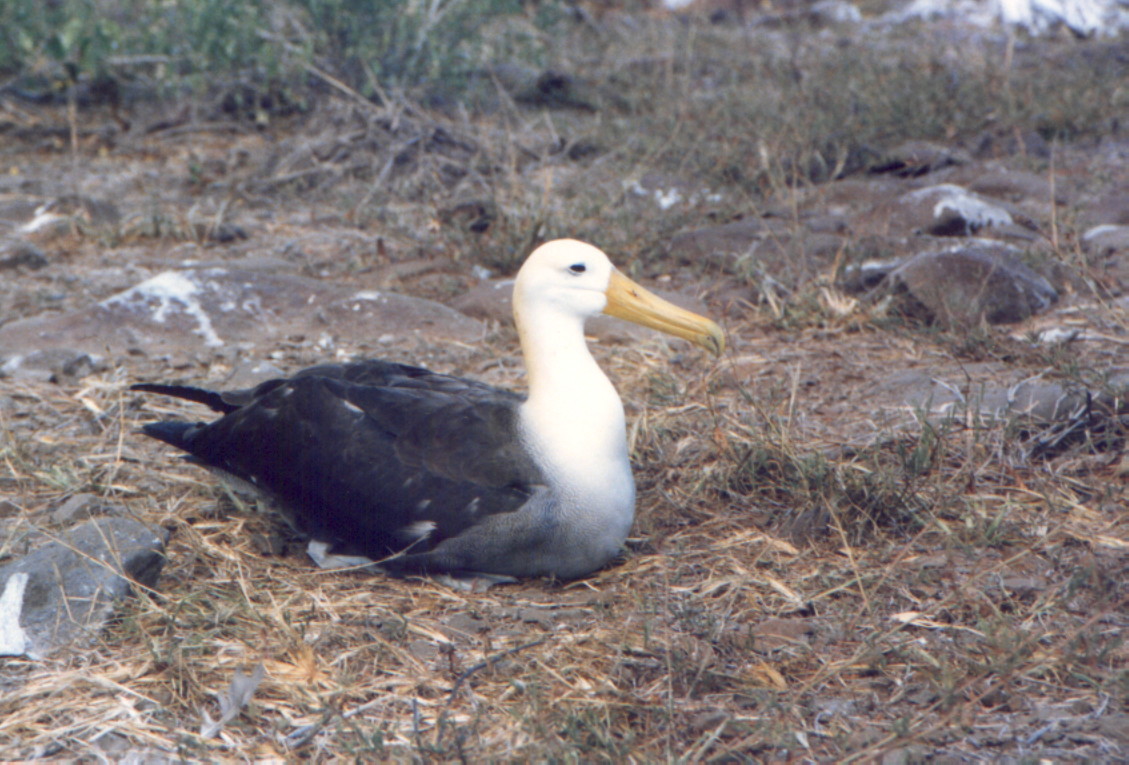The image depicts a seabird, possibly a seagull or pelican, resting on a patch of dry, dead grass interspersed with rocks. The close-up photograph captures the bird in profile, revealing its distinct white head and neck, along with a long, sharp yellow beak. The bird's body features black feathers with a gray belly. It appears tranquil as it looks out to the side, not facing the camera. The ground around the bird is a mix of dead grass, dirt, and rocks, with some patches of greener grass visible in the background. The overall setting is outdoors and gives an impression of a serene, yet somewhat rugged natural environment.